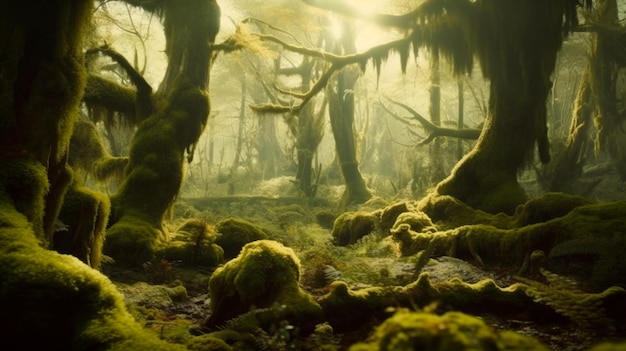The image depicts a lush, enchanting forest scene, either a photograph or a highly realistic animated style drawing. The forest is densely populated with at least ten trees prominently in the foreground, each cloaked in vibrant green moss, lending it a mystical, almost "Fern Gully" rainforest-like atmosphere. The trees' branches are adorned with wispy, hanging moss that gives an ethereal touch as if unraveling delicate threads. The ground is uneven, covered with rocks and roots, all blanketed in the same verdant moss, adding to the rich texture of the scene. In the center, an opening in the canopy allows sunlight to filter through, creating a hazy, dreamlike quality as it illuminates the moss-covered branches. The left side of the image features a particularly large tree, its base shrouded in darkness, while the right side also shows another significant tree and more greenery in the background. The depth of the forest is evident as the trees recede into the distance, cloaked in dark and light green foliage, enhancing the sense of mystery and endless natural beauty.